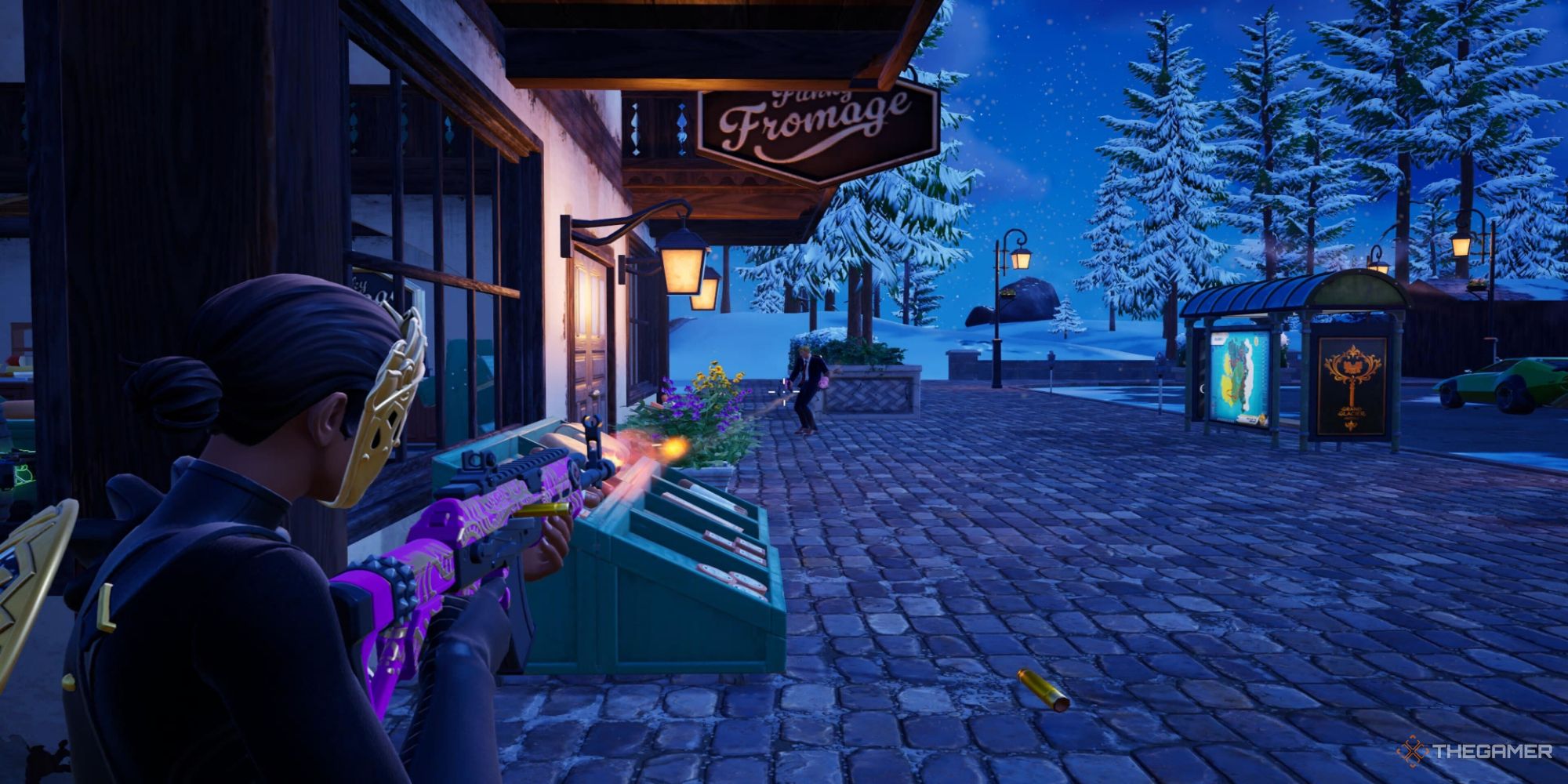The image is a detailed screenshot from a game, likely Fortnite, set in a snowy, nighttime village scene. The environment features cobblestone streets, a quaint shop with a sign that reads "fromage," and evergreen trees dusted with snow. In the immediate foreground, on the left, a woman stands in a full-body black suit and a gold face mask. Her hair is styled in a bun. She is aiming a violet-pink assault rifle with a black magazine, muzzle, and possibly a scope. An orange muzzle flash indicates she is actively firing the weapon. Bullet casings are being ejected, and she is aiming at a man in the distance, dressed in a suit with something pink visible on his body. This man stands near a shop that has dark brown wood and white-painted sections, reminiscent of stucco or plaster. The ground is covered in stone pavers, and there are vintage streetlights illuminating the scene. To the right, additional village elements include a green car, a bus stop, and green bins, which could be trash cans. The overall ambiance is serene yet tense, amplified by the starry sky and lightly falling snow. A watermark in the bottom-right corner reads "the gamer."